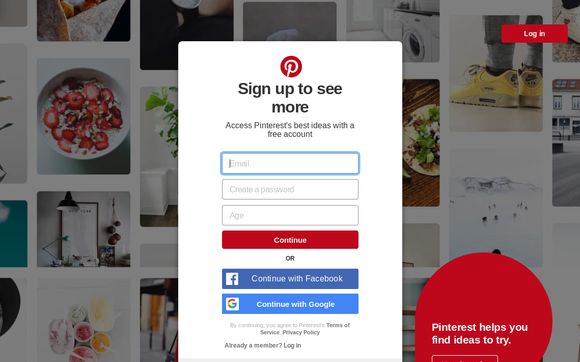This image is a cropped screenshot of the Pinterest sign-up page, prominently featuring a central white rectangular pop-up box against a background collage of various image pins, showcasing themes such as food, fashion, home décor, and products. 

At the very top center of the pop-up box is the Pinterest logo. Directly below this, bold black text reads "Sign up to see more." The following line, in smaller black font, states, "Access Pinterest's best ideas with a free account." The form below these instructions includes text boxes labeled for email, password, and age.

Beneath the form fields is a red button labeled "Continue." Further down, the word "or" is centered in capitalized bold black letters. The sign-up options continue with a button featuring the Facebook logo labeled "Continue with Facebook" and another button with the Google logo labeled "Continue with Google."

At the bottom of the pop-up box, smaller black text provides hyperlinked privacy policy and terms of service information. Additionally, a message reads, "Already a member? Log in," with "Log in" hyperlinked. For existing members, there's also a red "Log in" button at the top right of the screen with white text.

Finally, in the bottom right corner of the image, a red bubble includes the text "Pinterest helps you find ideas to try."